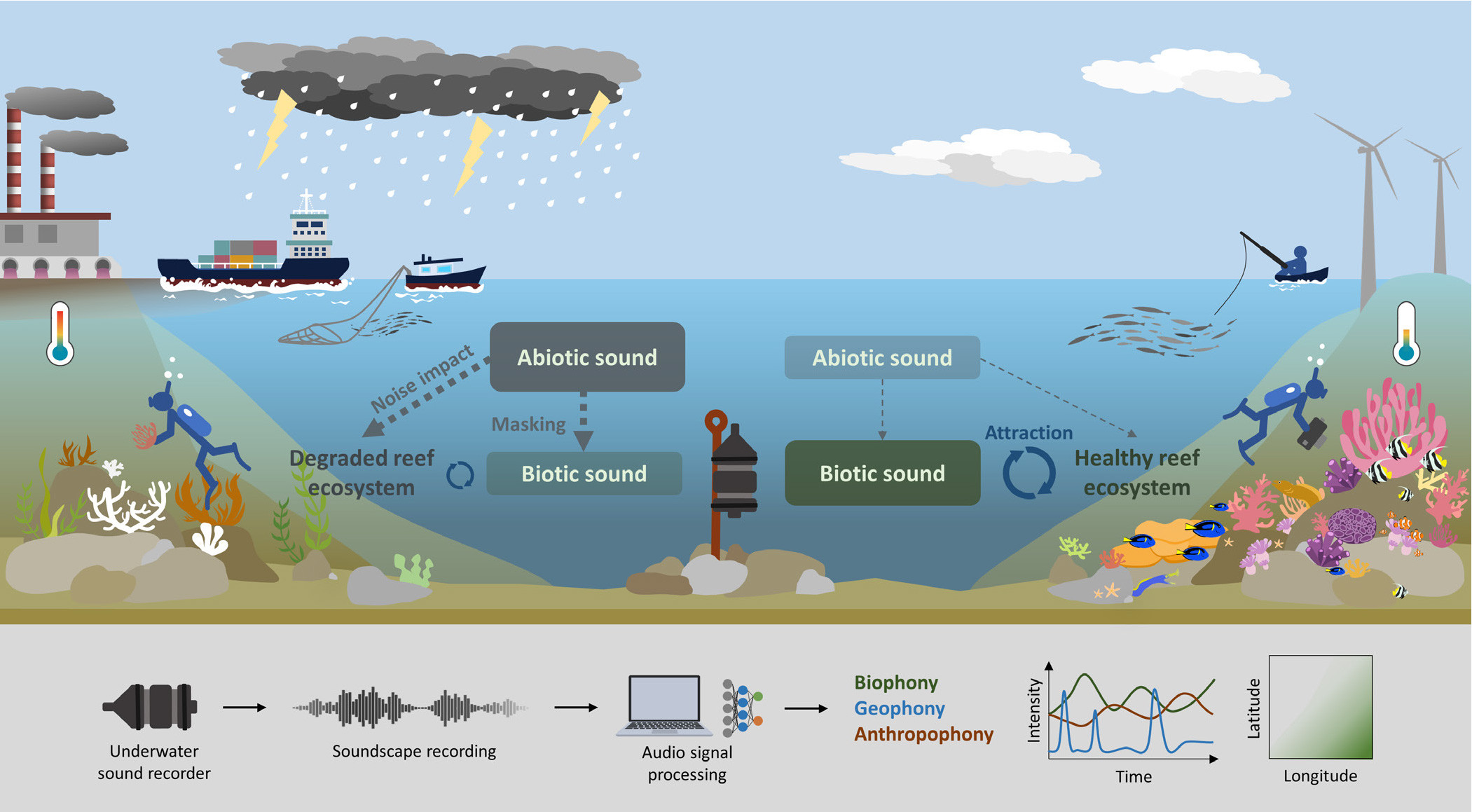The image is a rectangular scientific illustration, approximately six inches wide and three inches tall, depicting an oceanic sound system and ecosystem contrast. The top third of the image displays a sky scene from left to right, featuring a factory emitting gray smoke, a thundercloud releasing lightning and rain over two ships, white clouds, a wind farm, and fishermen on the sea. The middle section provides a side view of the underwater scene, showing a scuba diver, and differentiates between a degraded reef ecosystem and a healthy reef ecosystem. Labels such as "abiotic sound" and "biotic sound" direct attention downward, pinpointing areas labeled "noise impact" and highlighting the impact on reef ecosystems. The bottom section presents a gray background with a sequence of labels: "underwater sound recorder," "soundscape recording," "audio signal processing," and culminating in a graph with "biophony," "geophony," and "anthropophony." This graph illustrates sound intensity over time, with axes labeled for latitude and longitude in the lower right corner. The detailed elements enhance the visual comparison of degraded versus healthy ecosystems through the depicted sounds, interactions, and effects.